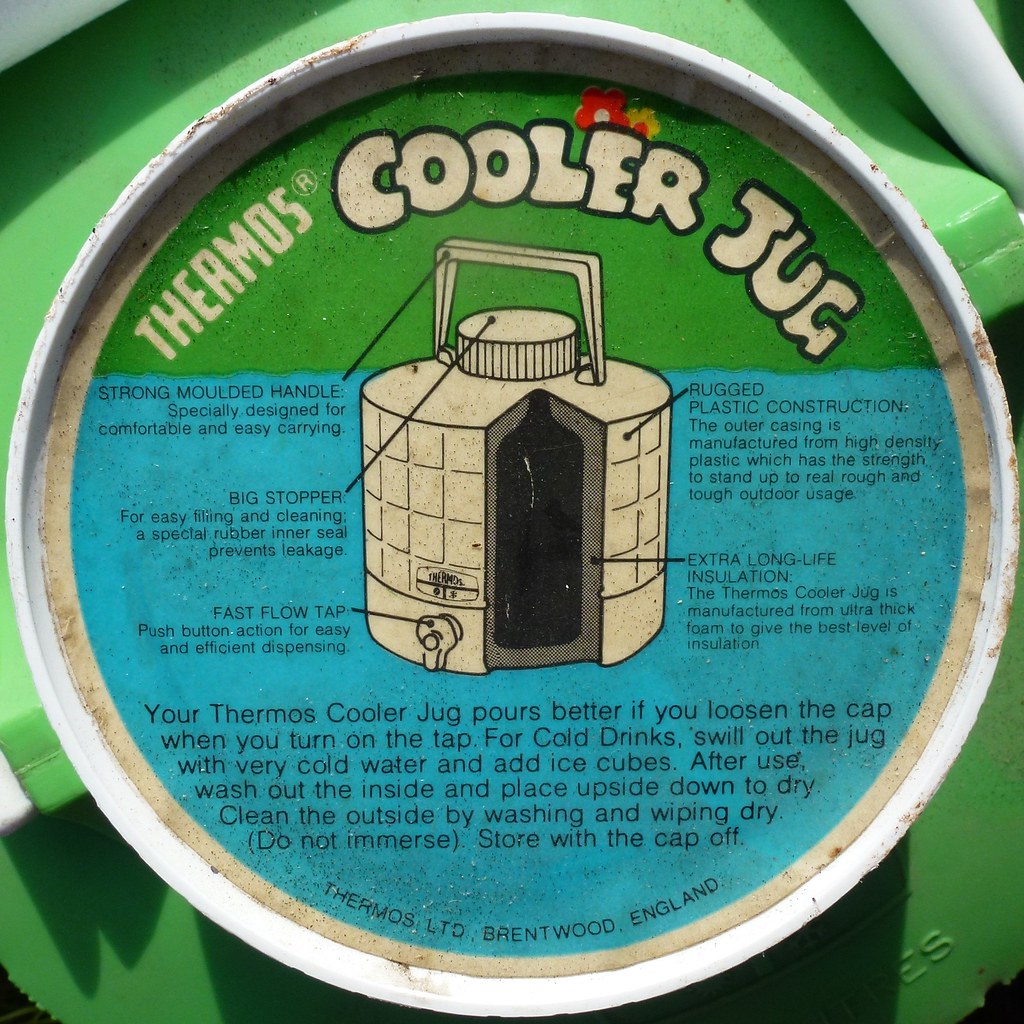The image showcases the top of a vintage Thermos cooler jug, with a worn, round sticker affixed to its lime-green screw top. The top third of the sticker is green, featuring the word "Thermos" in bubbly, white uppercase letters, complete with a registered trademark symbol. Below, in similarly styled white letters outlined in black, is the phrase "cooler jug." Red flower illustrations adorn the sticker, adding a touch of vintage charm. The sticker also includes detailed diagrams labeling parts of the jug, such as the strong molded handle, big stopper, fast flow tap, rugged plastic construction, and extra long life insulation. Surrounding these diagrams are instructions for optimal use and maintenance, advising to loosen the cap when pouring, swill with cold water and add ice cubes for cold drinks, wash and dry inside and out, and avoid immersion while storing with the cap off. The white handle attached to the jug contrasts with the green background, and the metal top shows signs of age, such as rust spots, reinforcing the nostalgic appearance of this classic cooler jug.